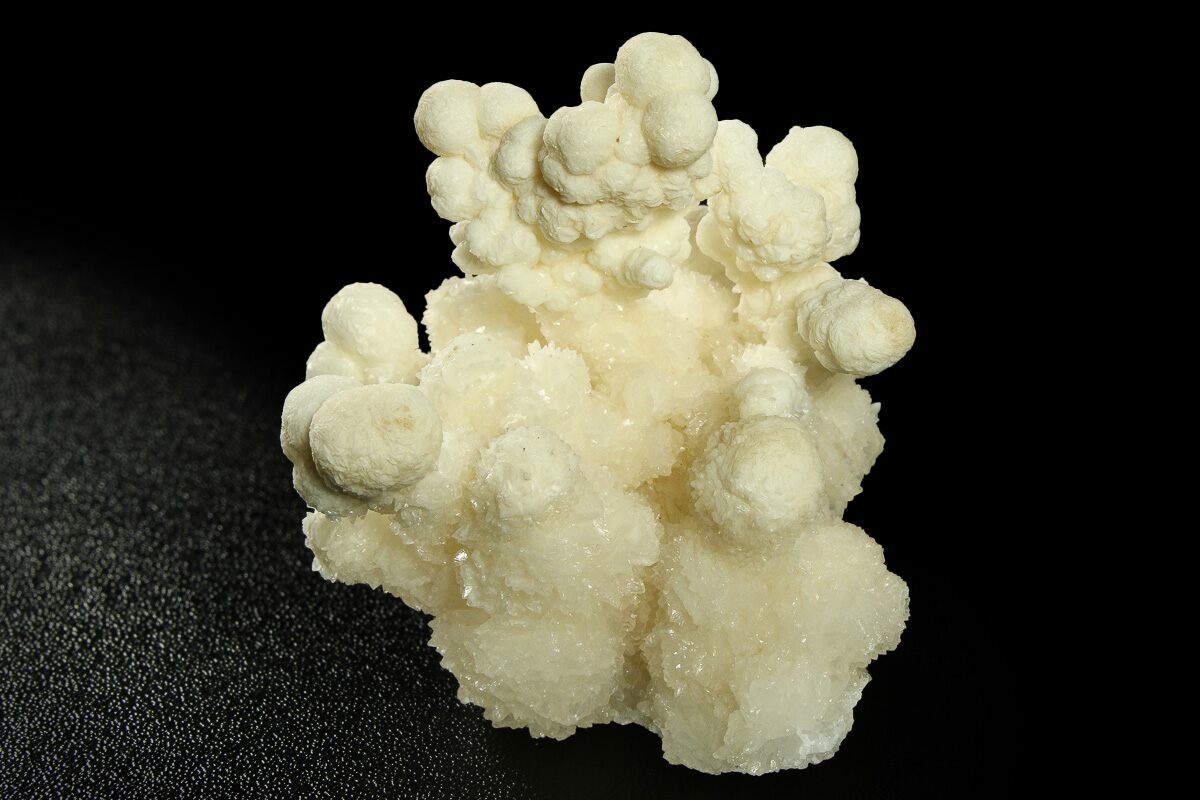The image showcases an intriguing off-white beige crystal resting on a black mat. The crystal is more heavily crystallized at its base, where the off-white color deepens slightly, adding contrast and highlighting the intricate crystalline structures sprouting from the bottom. Light reflects off the crystal, accentuating its textured surface. The upper part of the specimen is smoother and rounded, adorned with small, round nodules protruding from its sides and top. These nodular formations give the appearance of fluffy clouds settled on a mineral, adding a whimsical element to the otherwise rigid crystal. The contrast between the crystallized base and the rounded, nodule-covered top emphasizes the unique formation of this captivating mineral specimen.